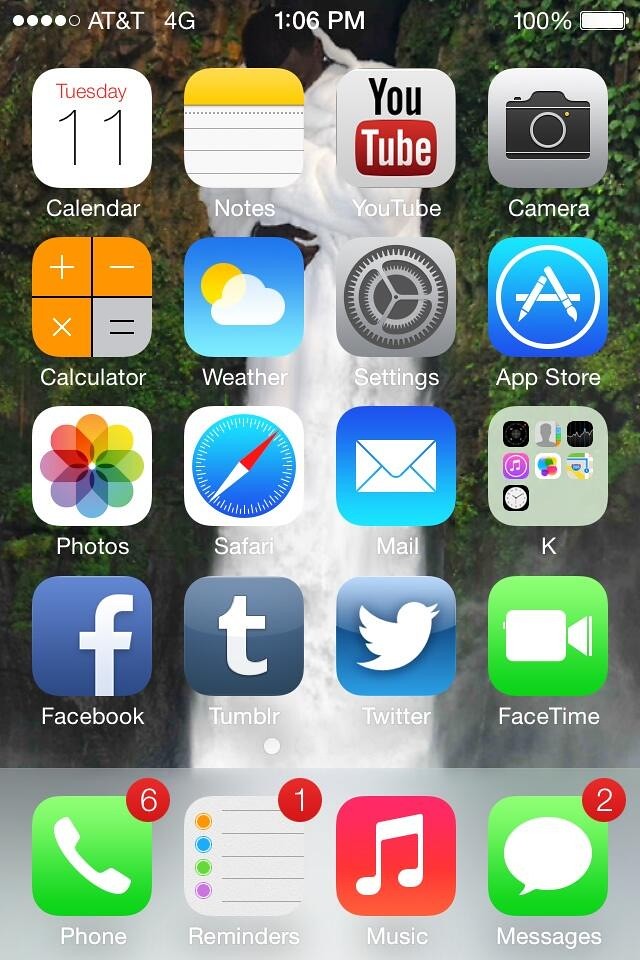A detailed screenshot of a phone screen shows the user connected to AT&T 4G, with the time displayed as 1:06 PM and the battery fully charged at 100%. The date is Tuesday the 11th, though the specific month is not indicated. The home screen is organized with a background image of a picturesque waterfall cascading down the center, flanked by rocks and lush trees on either side.

The top app displayed is the Calendar, followed by the Notes app and an old version of the YouTube logo. Below these, the Camera, Calculator, Weather, Settings, App Store, Photos, Safari, and Mail apps are neatly arranged. 

In one cluster named "K," the screen reveals apps including Game Center, Stocks, Maps, Contacts, iTunes, and Clock.

The bottom row features social media and communication apps including Facebook, Tumblr, Twitter, and FaceTime. The dock at the bottom houses Phone, Reminders, Music, and Messages apps.

Notification badges indicate two unread messages, six missed calls, and one pending reminder. The other apps are free of notifications. The screenshot captures the first page of the user's home screen, suggesting there could be additional apps on secondary pages.